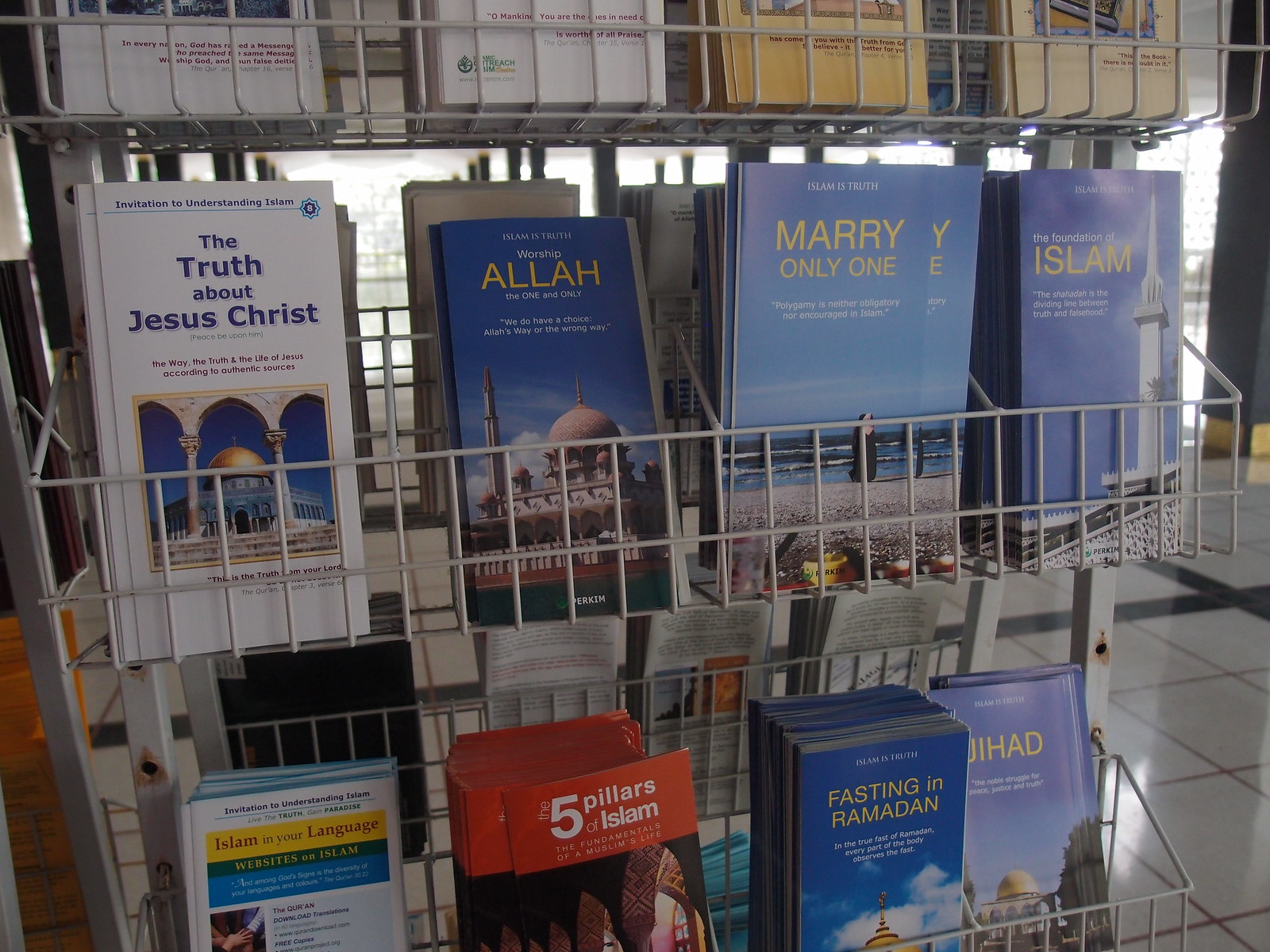This image captures a white wireframe brochure stand filled with an array of religious pamphlets, each offering insights into various aspects of Islam. The top row of pamphlets includes detailed topics such as "The Truth about Jesus Christ," which explores Jesus's life according to authentic sources and features an image of a mosque. Another pamphlet, titled "Islam is Truth: Worship Allah," emphasizes the singular worship of Allah and also showcases a mosque. A third brochure, "Marry Only One," discusses the stance on polygamy in Islam, accompanied by an image of a woman in a hijab or burqa walking on a beach. The fourth pamphlet on the top row, "The Foundation of Islam," highlights the importance of the Shahada with another mosque image. 

Below, additional brochures cover "Islam in Your Language" with information on related websites, "The Five Pillars of Islam," summarizing the core principles of Muslim life, "Islam is Truth: Fasting in Ramadan," detailing the comprehensive nature of the Ramadan fast, and lastly, "Islam, the Truth: Jihad," which defines Jihad as a noble struggle for peace, justice, and truth. The stand is set on a white-tiled floor, and in the background, through a window, parts of a cityscape are faintly visible, lending a subtle urban context to the scene.